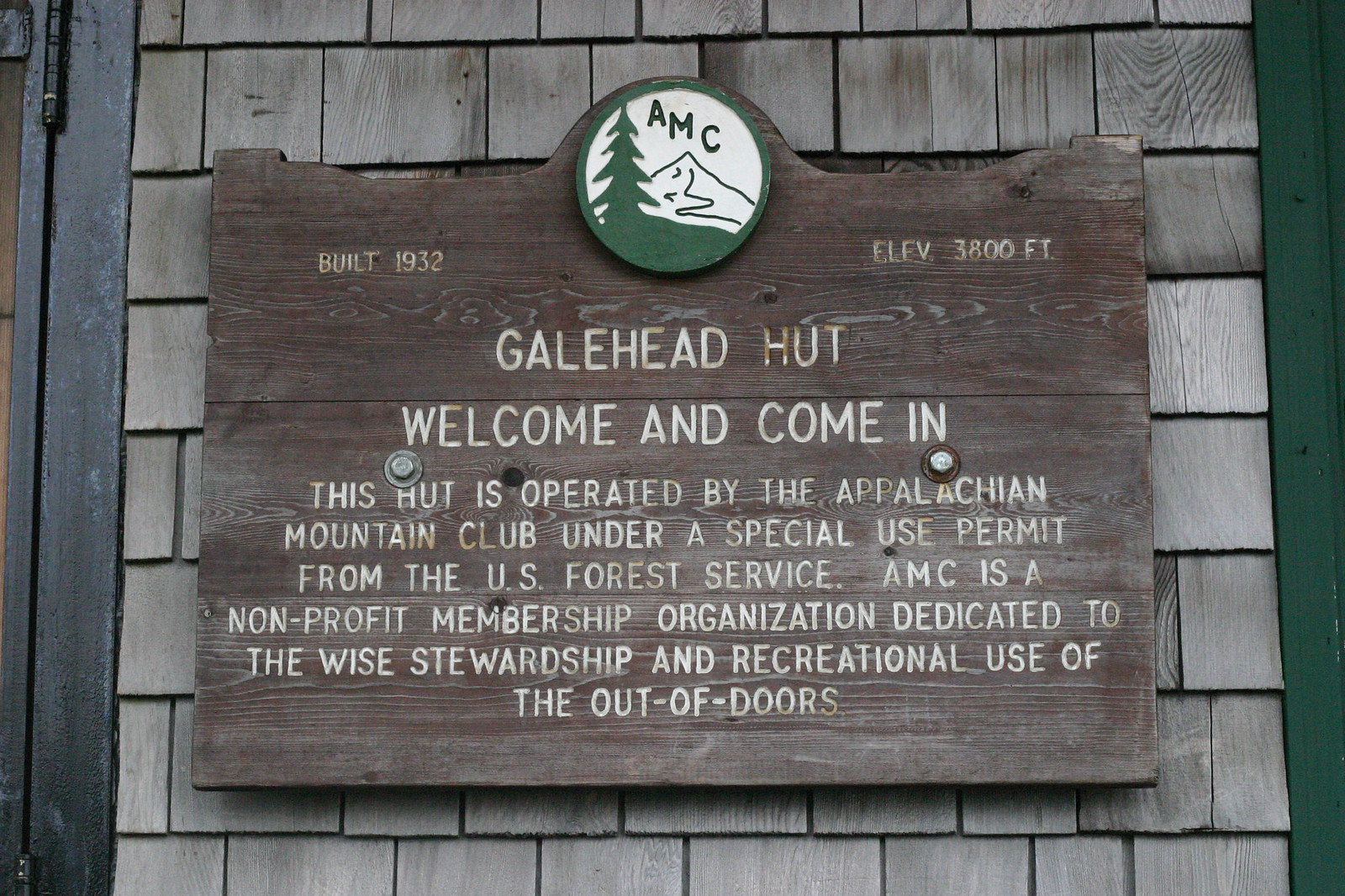The image features an exterior view of a building covered in cedar shakes with two doorways framed in dark green and black borders on either side. Prominently centered is a nearly square wooden plaque with an elaborate design. At the top of the plaque is a green-bordered circle featuring a white depiction of a pine tree alongside a mountain range, with "AMC" inscribed in green lettering above it. To the left of the circle, in tan writing, it says "Built 1932," and to the right, "Elevation 3,800 feet." The main section of the plaque, written in white, reads: "Gale Head Hut, welcome and come in." Further down, it states that the hut is operated by the Appalachian Mountain Club under a special use permit from the U.S. Forest Service. The AMC is described as a non-profit membership organization dedicated to the wise stewardship and recreational use of the outdoors. The plaque exhibits symmetry with centered text throughout, adding to the rustic charm of the setting.